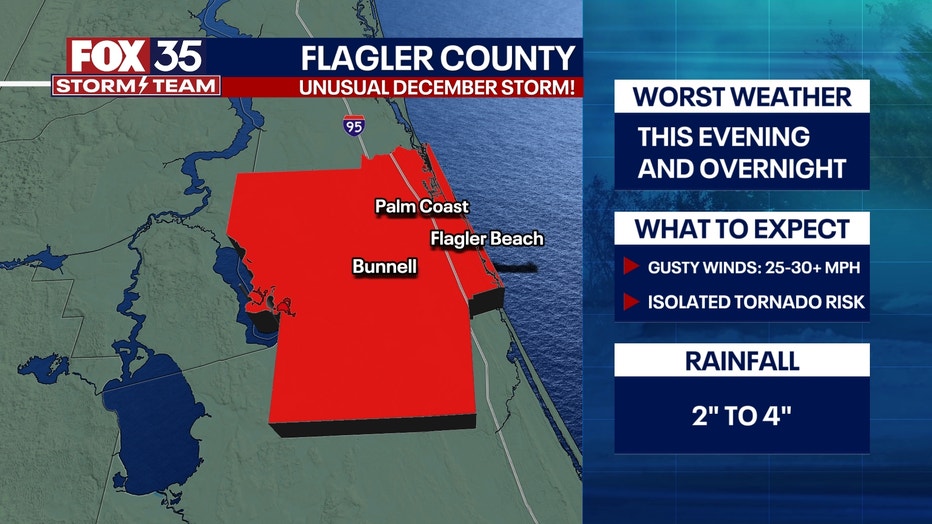The image is a screenshot of a weather forecast from the local news station, Fox 35. It shows a digital map of Flagler County, labeled as an unusual December storm. The map features a highlighted red area, indicating Palm Coast, Flagler Beach, and Bunnell. The left side of the map depicts the coastline with a calm sea, while the rest of the map is mostly green. A major route, I-95, runs parallel to the coastline. On the right side, there are vertical blue boxes with white headings, providing detailed weather alerts. The headings read: "Worst weather this evening and overnight," "What to expect: gusty winds 25 to 30+ mph," "Isolated tornado risk," and "Rainfall 2 to 4 inches." At the top of the image, a banner reads, "Fox 35 Storm Team, Flagler County, Unusual December Storm."